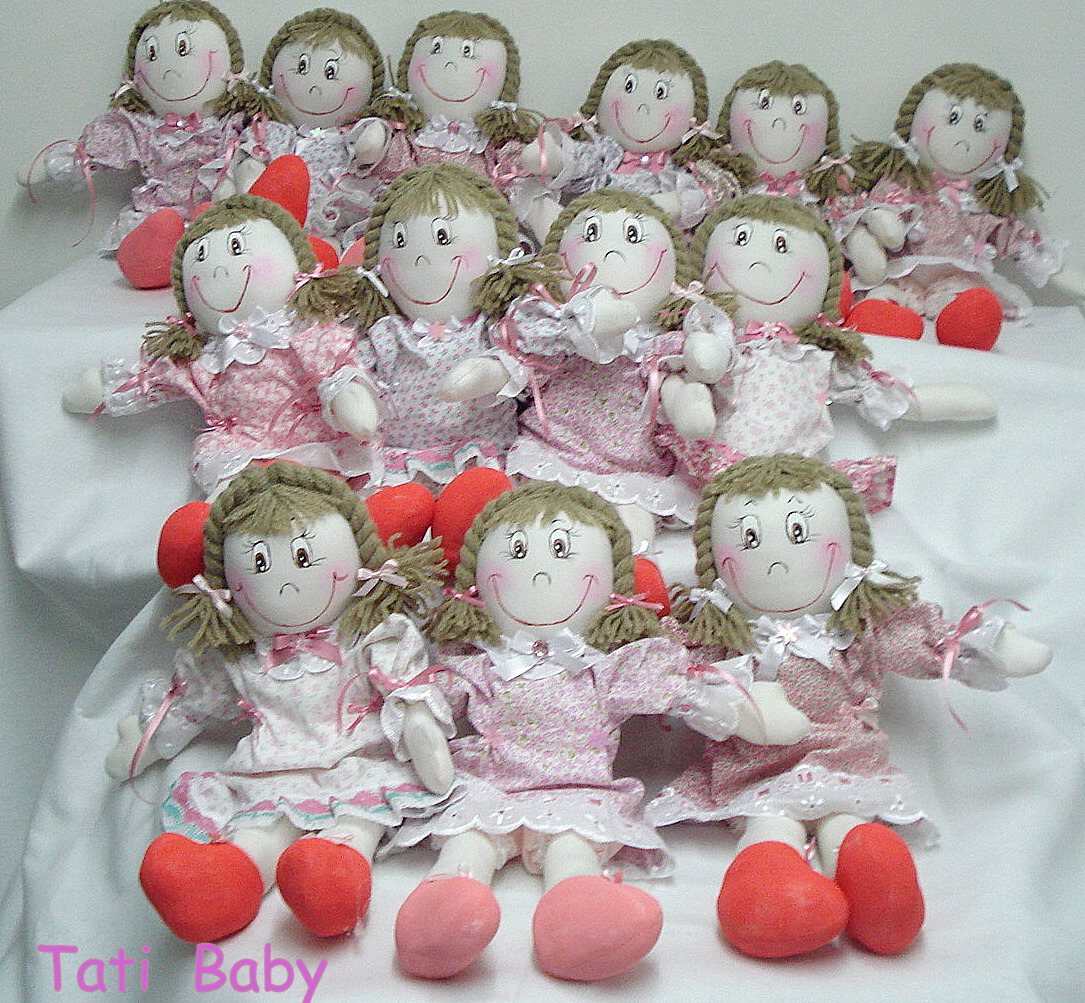The indoor photograph showcases three rows of nearly identical, handmade, all-cloth Raggedy Ann-type dolls, each with white fabric faces, small painted or embroidered black eyes, wide red smiles, rosy red cheeks, and narrow upside-down U-shaped noses. They feature yarn hair braided into two pigtails, adorned with either pink or white bows. Although their outfits differ slightly, all the dolls wear pink and white dresses with lace and ribbon details, featuring varied pink and white patterns. Some dolls wear pink booties while others sport orange or red ones. The dolls are meticulously arranged on a white sheet against a white wall, with six dolls in the back row, four in the middle row, and three in the front row. The bottom left corner of the photo features hot pink text in what appears to be Comic Sans font, reading "Tati Baby" (T-A-T-I B-A-B-Y).